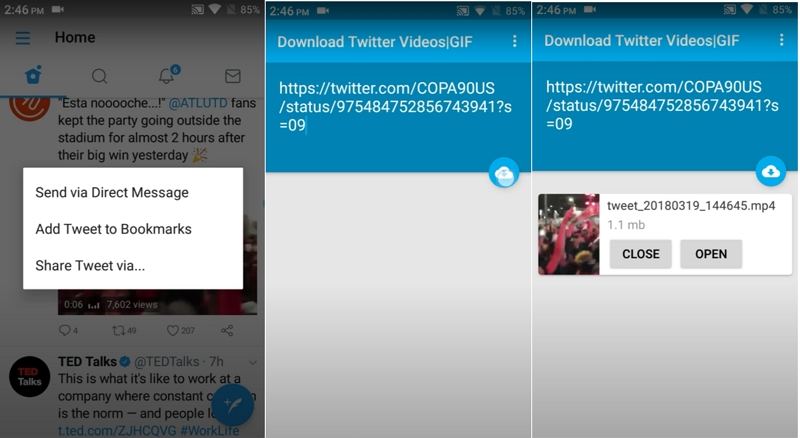This horizontal image, viewed on a smartphone, captures a busy screen filled with various icons and text, divided into three distinct vertical sections. 

In the upper-left corner of the first section, the time is displayed as 2:46 p.m. in white, next to a small video camera icon. On the opposite side, icons for Wi-Fi strength and a critically low battery (approximately 5%) are visible. Below the time, there are three horizontal blue lines, followed by the word "Home" in bold black text, and a house icon. Adjacent to these, there is a magnifying glass icon, a bell icon indicating six notifications, a mail symbol, and a partial view of a circular profile picture. 

Directly beneath, there's a tweet that reads, "Esta noche at altitude fans kept the party going outside the stadium for almost two hours after their big win yesterday," accompanied by a celebratory emoji. Below the tweet, there's a white box with options to "Send via Direct Message," "Add Tweets to Bookmarks," and "Share via Tweet."

The second section contains another tweet from TED Talks, mirrored by similar icons at the top. This section also features an option to "Download Twitter Video GIF" with an associated web address.

In the third section, the tweet again promotes "Download Twitter Video GIF" with a web link, and includes tweet details, mentioning a size of 1.1 MB. Options at the bottom allow the user to either close or open this section.